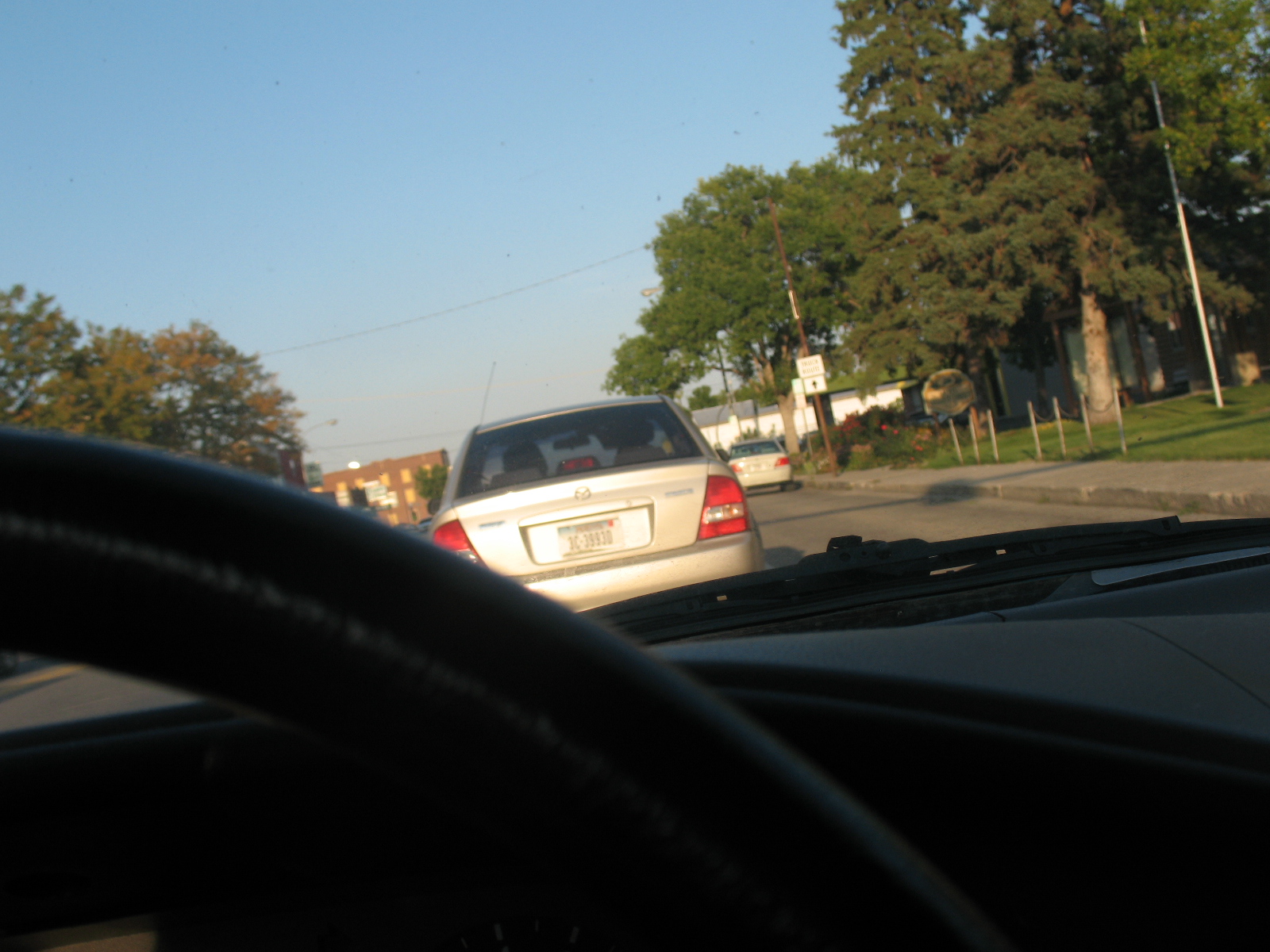The image is a landscape-oriented photograph captured from the viewpoint of a driver inside their car, during the daytime around 3 or 4 in the afternoon. The clear blue sky shows no clouds, though there seems to be some smog near the horizon. At the bottom of the picture, the dashboard and upper-right corner of the black steering wheel are visible, indicating the person might be taking the picture with their phone while driving. The windshield wipers can faintly be seen at the base of the windscreen, which has a slight glare. Directly ahead, in the lane in front, there's a silver or champagne-colored sedan, possibly a Mazda, with a license plate that is too blurred and glared by the sun to be readable. The road is flanked by trees on both sides, and to the right, there's a footpath, a grassy area, and what might be a park. The photo also captures power lines and the presence of other cars, suggesting a busy city scene. It appears they are either stuck in traffic or momentarily stationary.